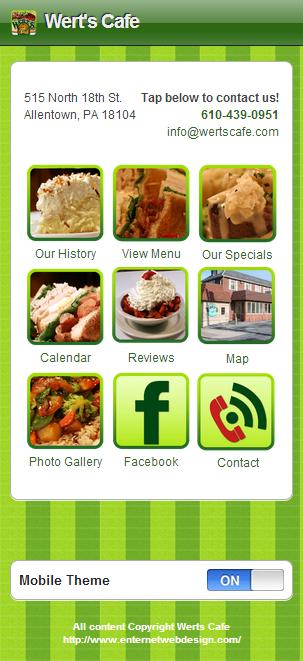This image is a screenshot of a mobile webpage for Wurtz Cafe, located at 515 North 18th Street, Allentown, Pennsylvania, 18104. The website features a green and white color scheme, with dark green and light green vertical stripes in the background, and a dark green border at the top. The name "Wurtz Cafe" is prominently displayed in white lettering on the dark green section.

Beneath the title, there's a large white rectangle containing the cafe's address, phone number (610-439-0951), and email (info@wurtzcafe.com), with a prompt to "Tap below to contact us."

Below this information are nine small icons arranged in a 3x3 grid, each with descriptive text and images. The icons include:
1. Our History – a slice of pie or cake.
2. View Menu – various food items.
3. Our Specials – more food images.
4. Calendar – image of food.
5. Reviews – image of food.
6. Map – a picture of a building.
7. Photo Gallery – images of food.
8. Facebook – a green Facebook logo.
9. Contact – a phone receiver icon.

At the bottom of the page, there's a white banner reading "Mobile theme on" with an on/off toggle switch set to "on," and some additional copyright information.